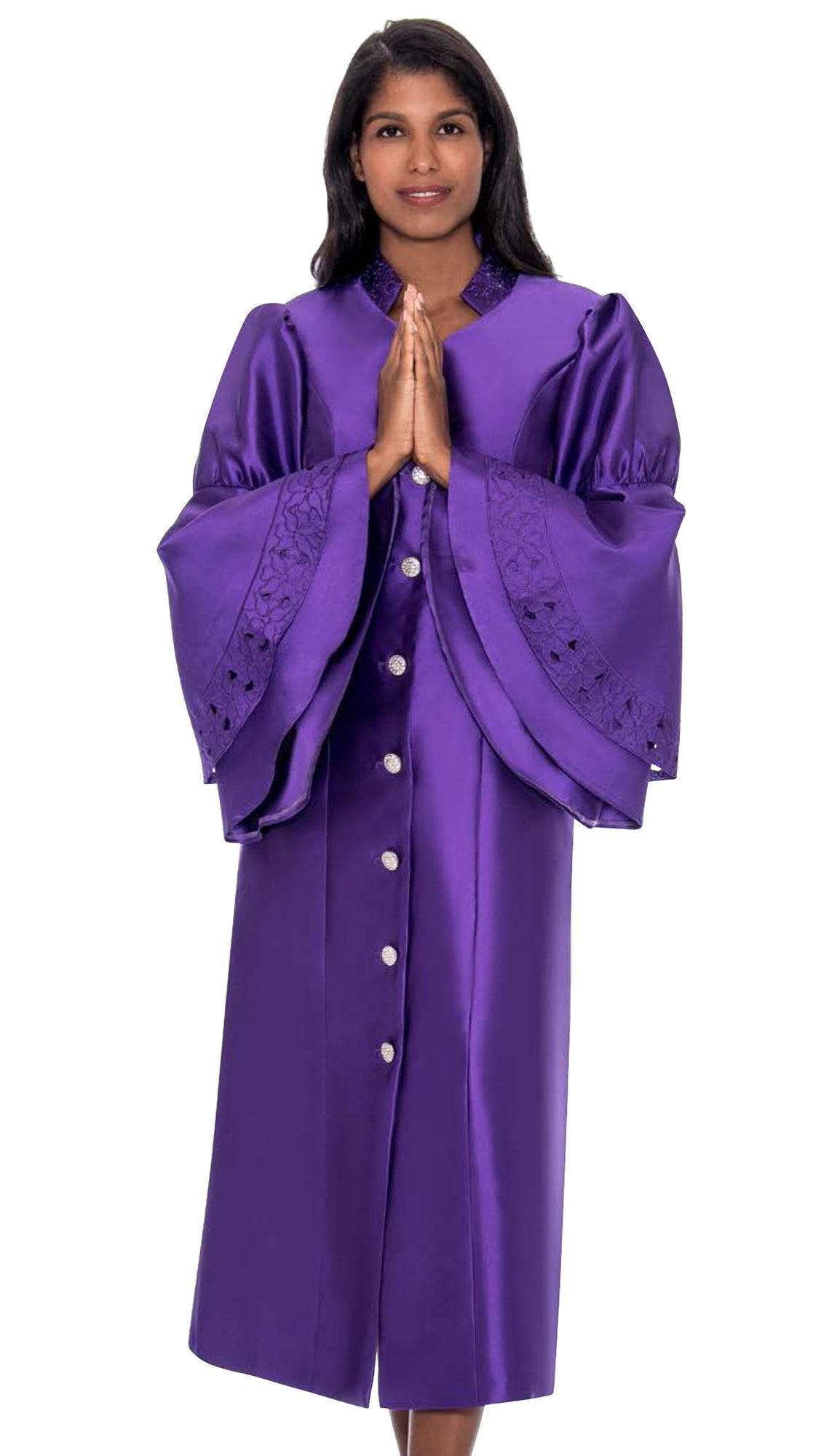This vertically oriented, realistic photograph showcases a young woman, possibly in her late teens or twenties, positioned against a pristine white background. Her caramel brown skin and luxurious, dark black hair, which cascades past her shoulders, add to her striking appearance. She is dressed in a long, silky, royal purple robe reminiscent of clerical attire, extending from her shoulders to her shins. The robe is adorned with silver buttons running down the center and features finely detailed open sleeves. The woman stands with her hands reverently folded together in a prayer-like pose, near her chest, and gazes directly at the viewer, exuding a sense of solemnity and grace.